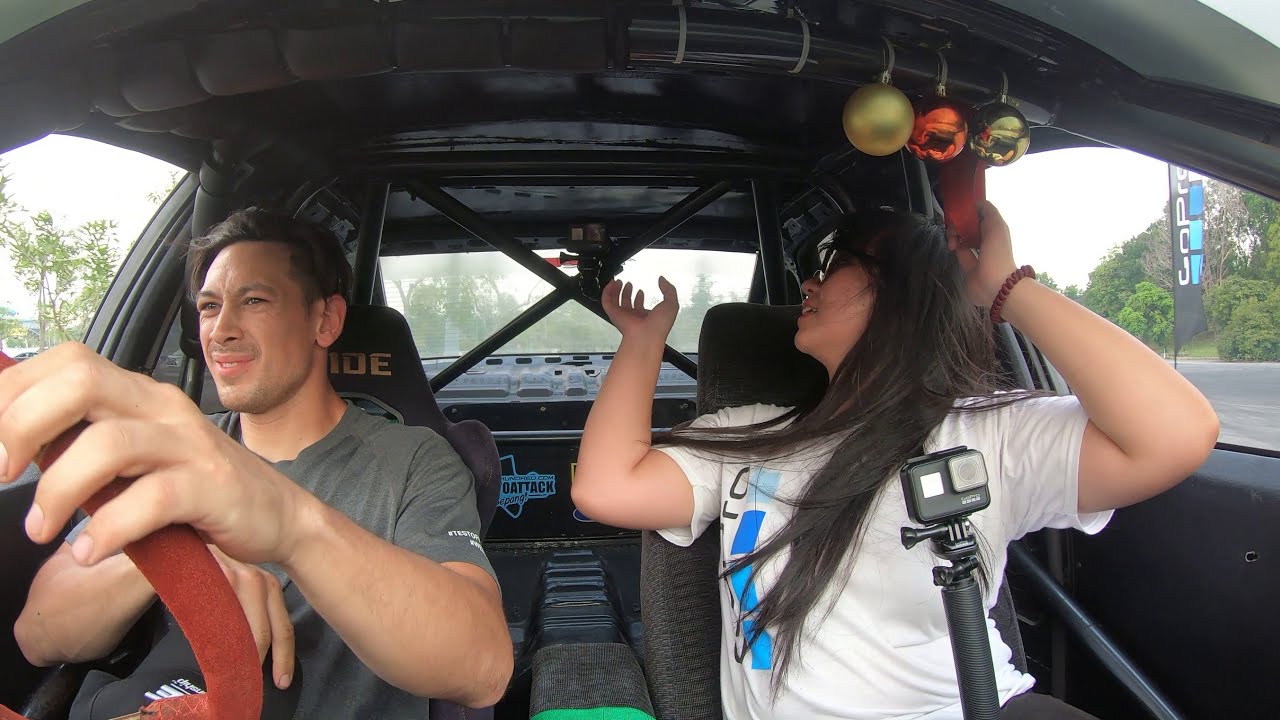In this photograph taken from the dashboard of a car, the camera captures the interior view, focusing on the driver and the passenger. The driver, an Asian man in his 20s with medium-length dark hair shaved on the sides, is wearing a grey t-shirt. He grips a distinctive red steering wheel with one hand while looking intently out the front windshield. Next to him, on the passenger side, sits a young Asian woman with long black hair, clad in a white t-shirt possibly featuring a GoPro logo on the left side. She holds a GoPro camera mounted on a small tripod in her lap and looks backwards over her right shoulder. The car's interior is predominantly black and features a roll cage, suggesting it could be a racing or derby car. Adding a festive touch, several colorful glass Christmas ornaments hang from the roll cage above the passengers' heads. Through the windows, the exterior view reveals a tranquil scene with trees and an empty road, indicating a day drive.